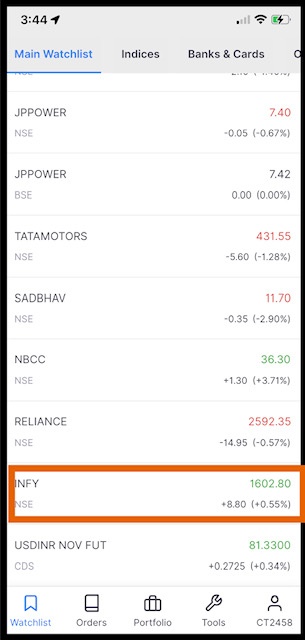A smartphone screen displaying a financial statistics website at 3:44 (unknown if AM or PM). The phone has a low battery with less than half remaining, weak cellular signal with only one bar, but Wi-Fi is enabled. At the top, blue text reads "Main Watch List" which is underlined, followed by "Indices" and "Banks and Cards." Below that, the screen shows various stock entries:

- JP Power NSE: 7.4 (down 0.05 points)
- JP Power BSE: 7.42 (no change)
- Tata Motors NSE: 431.55 (down 5.6 points)
- SADBHAV: 11.7 (down 0.35 points)
- NBCC NSE: 36.3 (up 1.3 points, indicated in green)
- Reliance: 2592 (down 14.95 points, indicated in red)

All stock entries, except NBCC NSE, are shown in either black or red text indicating no change or decrease in value.